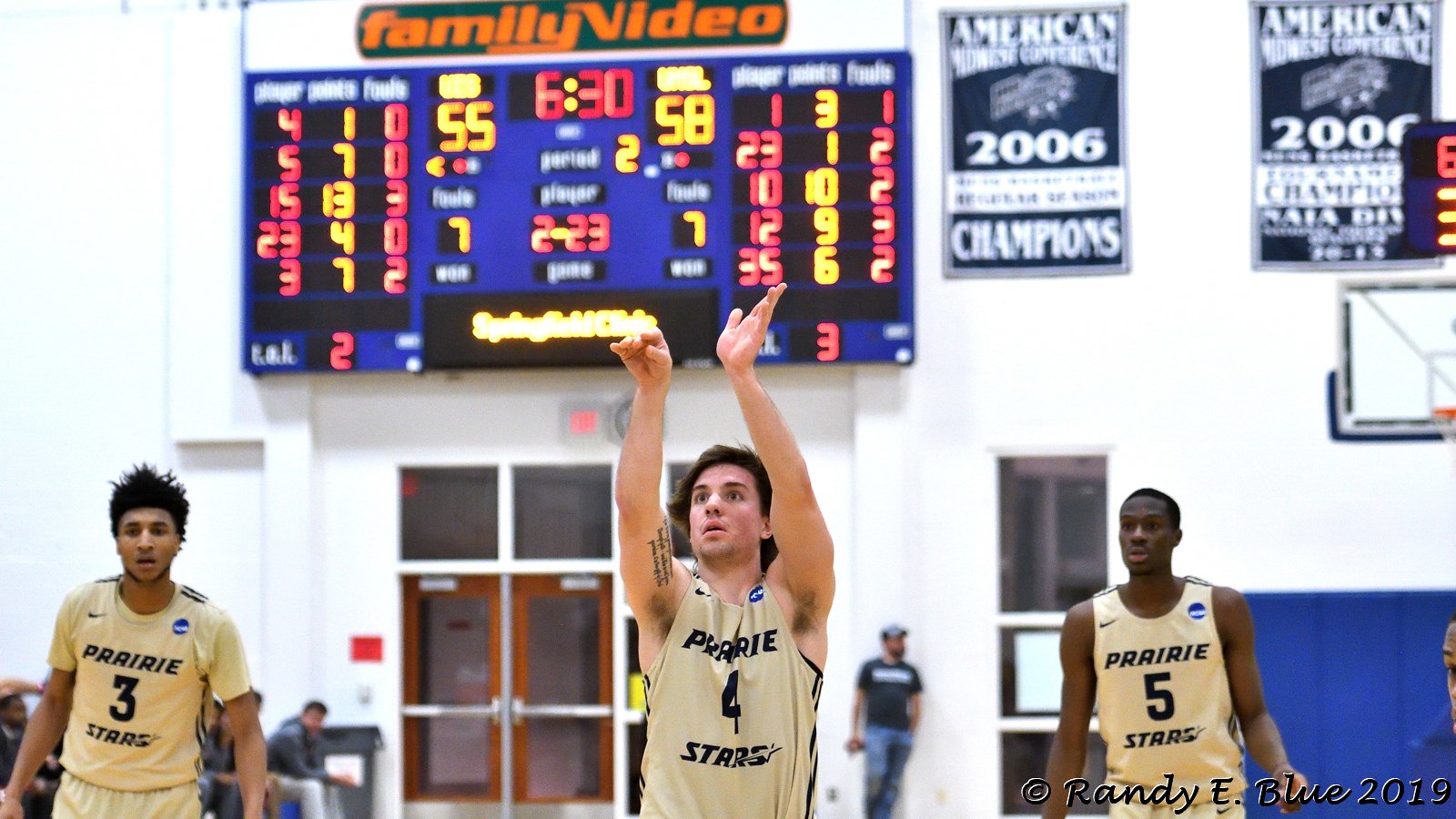This photograph captures an intense moment in a high school basketball game, featuring three young men in tan and black uniforms. The central player is captured mid-shot, his hands raised as he aims for the hoop, while his teammates on either side watch intently. Behind them, a large blue scoreboard dominates the gymnasium wall, showing a close game with one team at 55 points and the other at 58, with 6 minutes and 30 seconds left to play. Above the scoreboard, "Family Video" is prominently displayed. Flanking the scoreboard are banners, including a visible championship banner from 2006. In the background, some spectators stand near a double door, adding to the charged atmosphere of the game. The setting is further detailed with various posters, banners, and flyers adorning the wall, capturing the vibrant and communal spirit of this high school sports event.